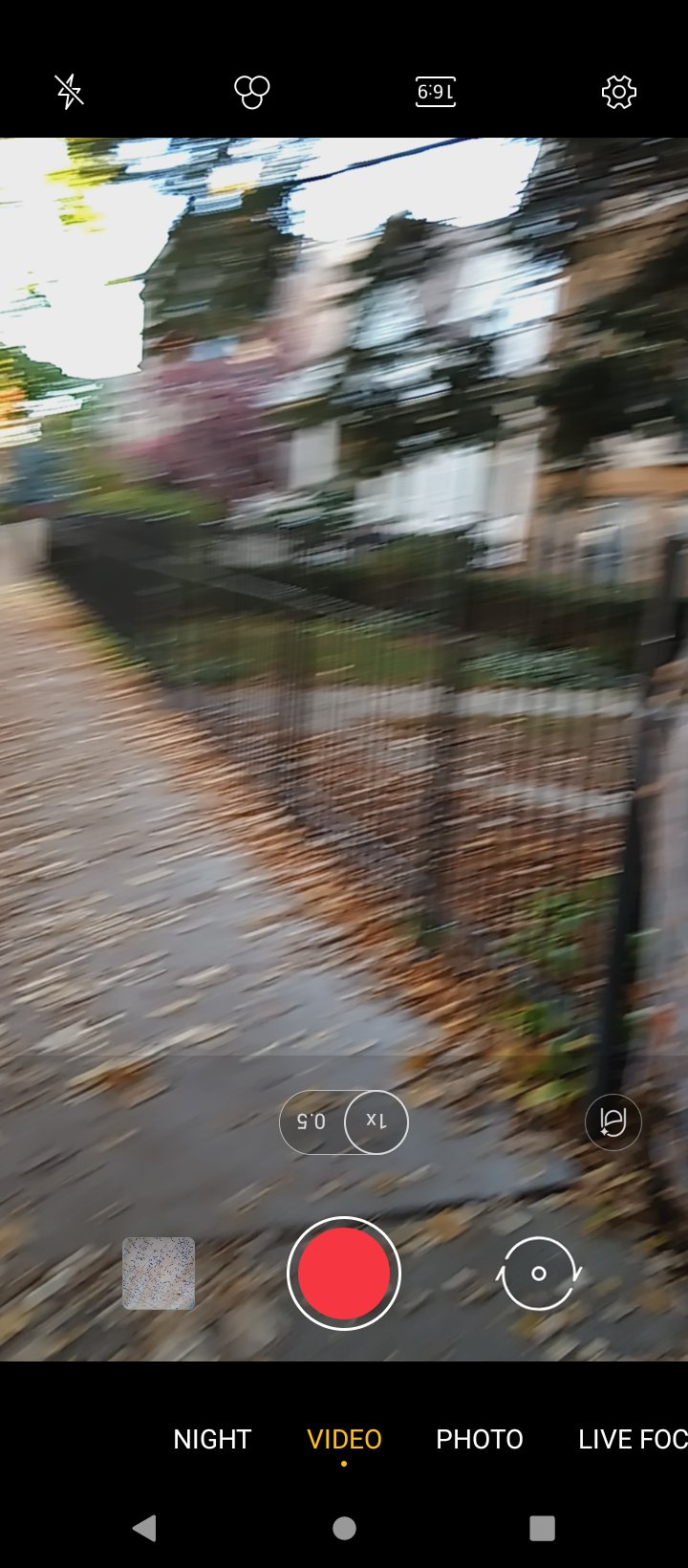This image is a detailed screenshot of a smartphone’s camera app interface, specifically on an Android device. The interface is displaying various camera mode options like 'Night', 'Video', 'Photo', and 'Live Focus', with the 'Video' mode highlighted in yellow, indicating the user's current selection. The screen includes the typical Android navigation bar at the bottom featuring the left arrow, circle, and square icons. The camera app's distinctive red record button with a white border is prominently visible, showing the device is ready to record but not actively recording. The main scene showcased through the camera depicts an autumnal residential neighborhood with several houses, black gates, and garden areas. Fallen brown leaves cover the ground, reinforcing the autumn season. There are also top and bottom black banners containing camera settings like exposure and flash. Interestingly, part of the text, particularly the zoom indicators '1x' and '0.5', appears inverted, suggesting the phone might be held upside down.